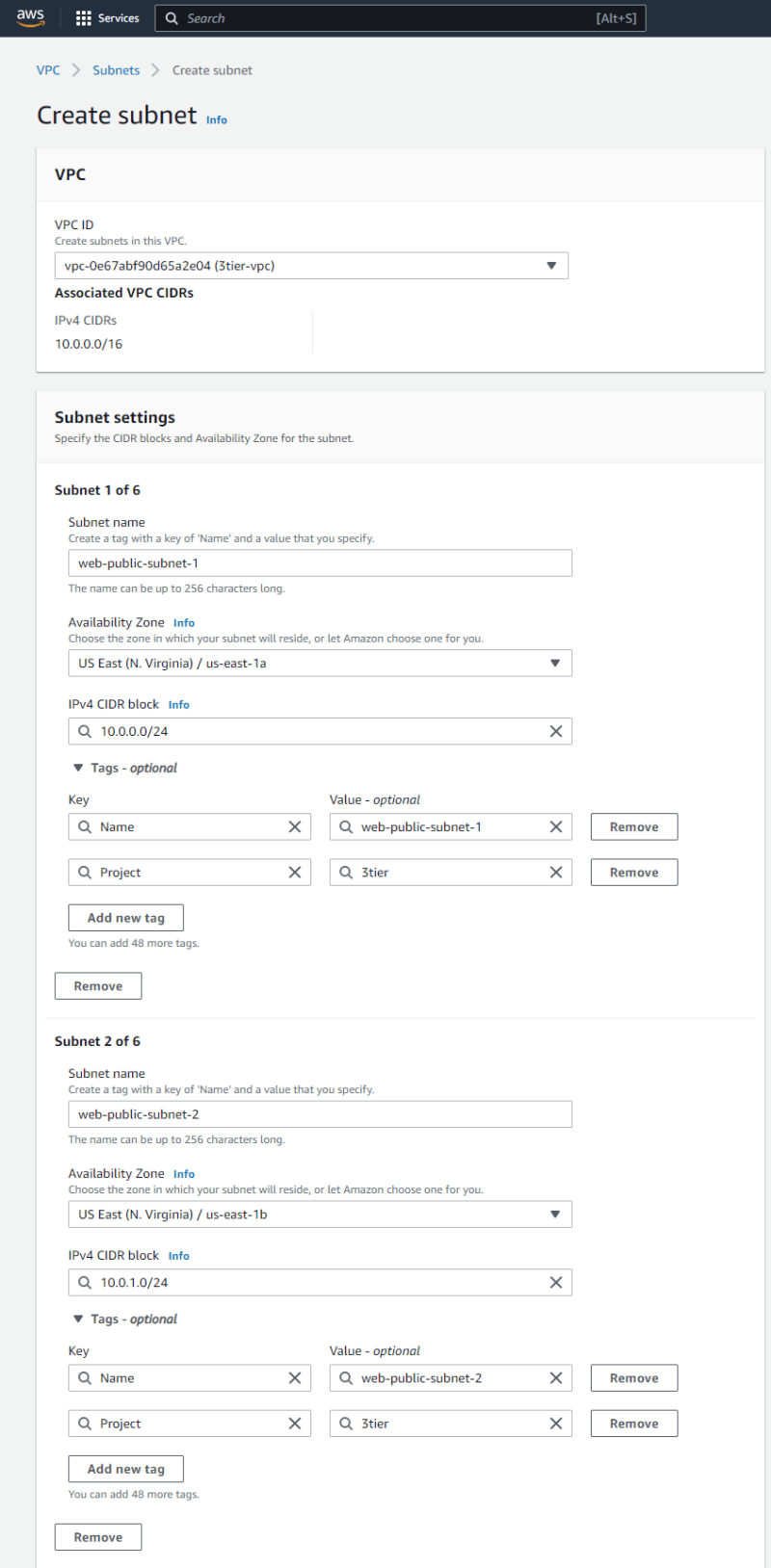This screenshot captures a mobile view of an Amazon Web Services (AWS) webpage focused on creating a subnet. 

In the upper left corner, there's a dark blue navigation bar featuring the AWS logo, which includes the signature yellow Amazon smile underneath. To the right of the logo, there is a clickable tab icon for services, represented by a grid of nine white square boxes arranged in three rows and three columns. Adjacent to the services tab is a search bar with a dark black background. The search bar, a long rectangle, includes a white magnifying glass icon next to the word "Search" and offers a keyboard shortcut (Alt + S) for quick access.

Beneath the navigation bar, a breadcrumb navigation trail is displayed, starting with "VPC," followed by "subnets," and ending with "create subnet," with each item separated by right-pointing arrows. The breadcrumb "create subnet" is highlighted or grayed out, indicating the current page. The overall title of the page is "Create Subnet," confirming that the user is on the section of the AWS website dedicated to subnet creation.